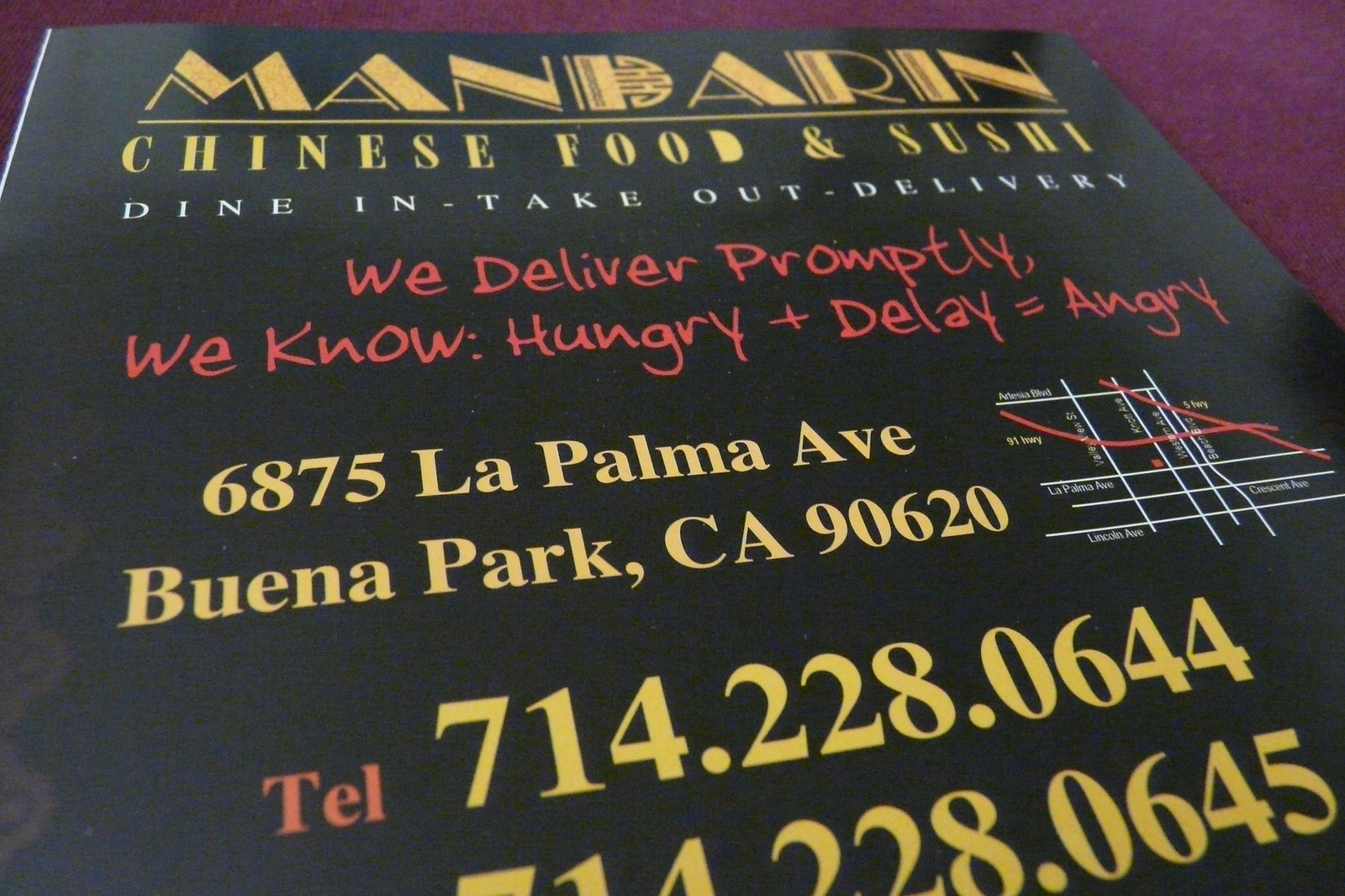In the image, a business card-sized advertisement for a Chinese food and sushi restaurant named "Mandarin" occupies the entirety of the frame, lying flat against a maroon or red surface, which could be a tablecloth. The background appears red, but there's a possibility of a purple hue. The ad's prominent text, written in yellow and white fonts with some artistic flair, announces "Mandarin, Chinese food and sushi." The card further details the dining options available: "Dine in, take out, delivery." Highlighting their fast delivery service, the ad humorously states, "We deliver promptly. We know. Hungry plus delay equals angry."

Below this, the address is listed in yellow: "6875 La Palma Avenue, Buena Park, California, 90620." Adjacent to the text, there is a small map displayed in white and red lines, indicating local streets and landmarks near the restaurant. Additionally, the ad provides two contact numbers in pink text: "TEL: 714-228-0644 and 714-228-0645." The overall setting of the image could either be indoors or outdoors, as the exact environment is ambiguous. The advertisement is primarily black with yellow, white, pink, and reddish accents, giving it a striking and vibrant appearance.